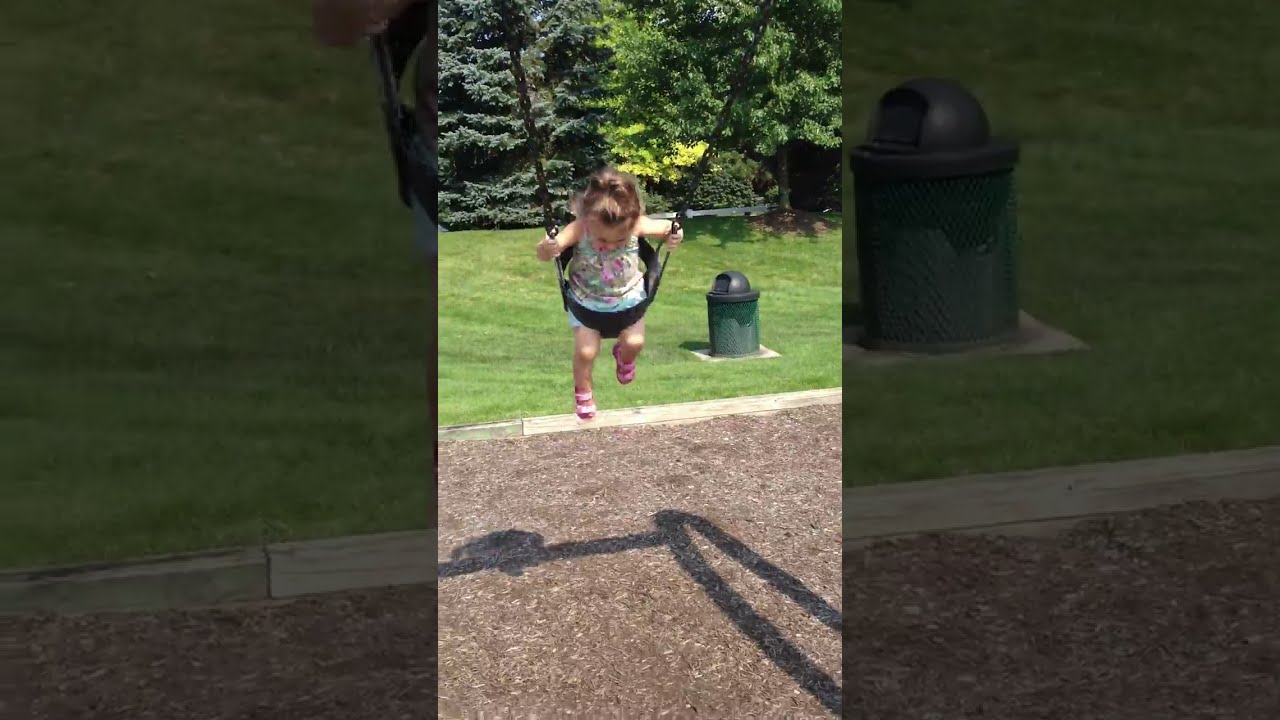This image vividly captures a joyful young girl, around three to four years old, with long brown hair tied in a ponytail, smiling widely and possibly laughing as she swings happily in a park. She is seated in a black swing designed with leg holes and suspended by dark metal chains. The ground beneath the swing is covered in mulch, thoughtfully laid for safety. The park setting is impeccably maintained, featuring freshly cut, green grass with visible mowing patterns. In the backdrop, tall evergreen and lighter green trees stretch up against a clear, blue sky. A green metal trash can with a gray lid is stationed to one side, completing the serene, picturesque scene. It's mid to late evening, suggested by the long shadows cast, adding a tranquil ambiance to the lively moment.